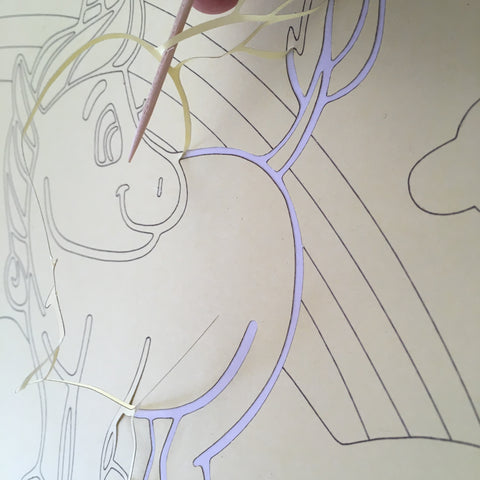The image showcases a hand-drawn, stenciled illustration of a unicorn, partially revealed through the peeling away of paper. The unicorn, facing left but glancing back to the right, is adorned with lines in a soft lilac hue, contrasting its primarily black and white form. It stands before an incomplete rainbow and a piece of a cloud to its right. A tool, resembling a thin spindle and likely pink, is being used to peel the paper, partially visible alongside the top of a finger at the image's upper edge. The scene suggests a whimsical, childlike artistic endeavor.